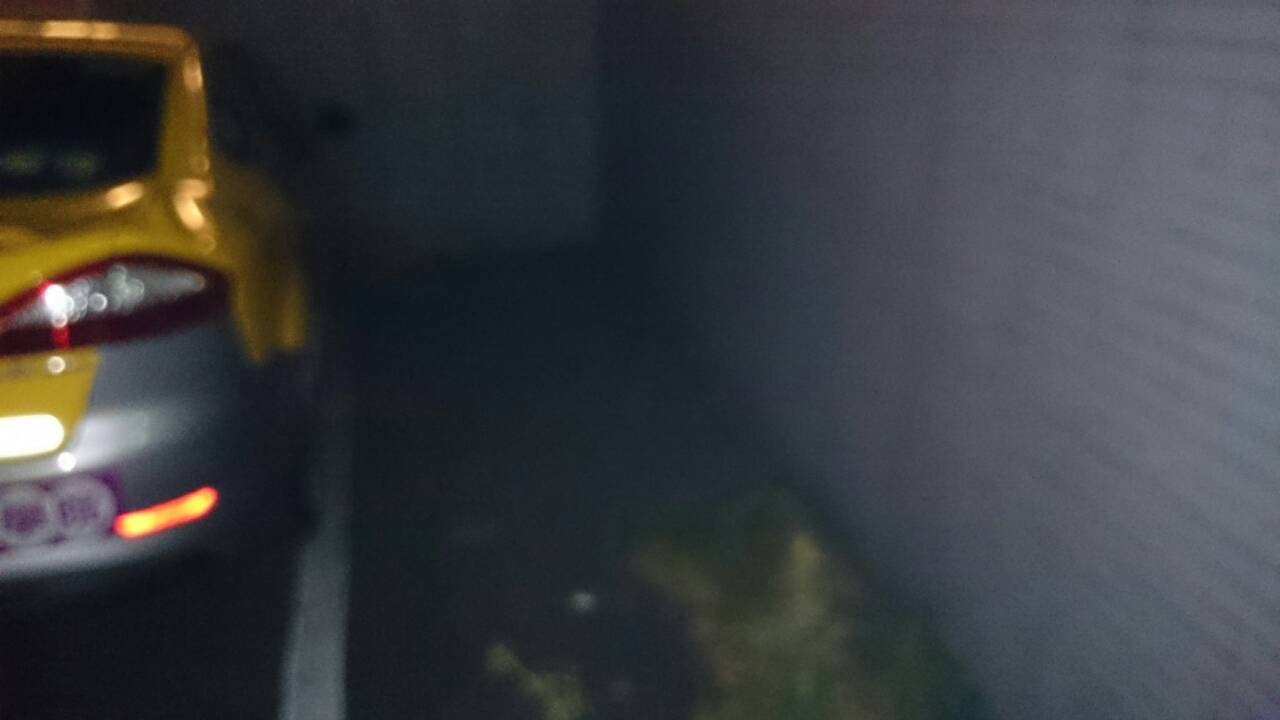The photograph depicts the rear view of a yellow and gold high-gloss car, likely a taxi, parked in a dimly lit, somewhat eerie garage. The setting includes a concrete floor with a white line extending from the back to the front of the car, indicating a pathway or division. A white or tiled wall stands to the right of the vehicle, with extra space between the car and wall potentially serving as a walking area. The image is quite blurry, and the dark, hazy ambiance is punctuated by the faint orange glow near the car's bumper. Stickers, possibly with Chinese writing, adorn the lower part of the car. In the foreground, an indeterminate, smudge-like artifact is visible on the ground, contributing to the overall unsettling feel of the space.